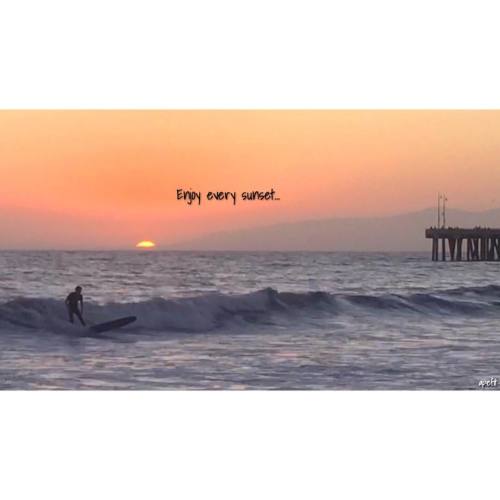The image features a captivating sunset scene over the ocean, characterized by an orange and pink sky. On the left side, a surfer stands upright on a surfboard, riding a small wave. The sun, barely visible with its top shaved off, is setting slightly left of center, casting a hazy orange hue across the horizon. A wooden pier supported by stilts extends from the right side into the mid-section of the photo. Above the sun, towards the center-left of the image, the black text reads "enjoy every sunset...". Additionally, there is small, somewhat difficult-to-read white text with a black shadow on the bottom right corner. The overall atmosphere suggests a serene and picturesque coastal sunset.